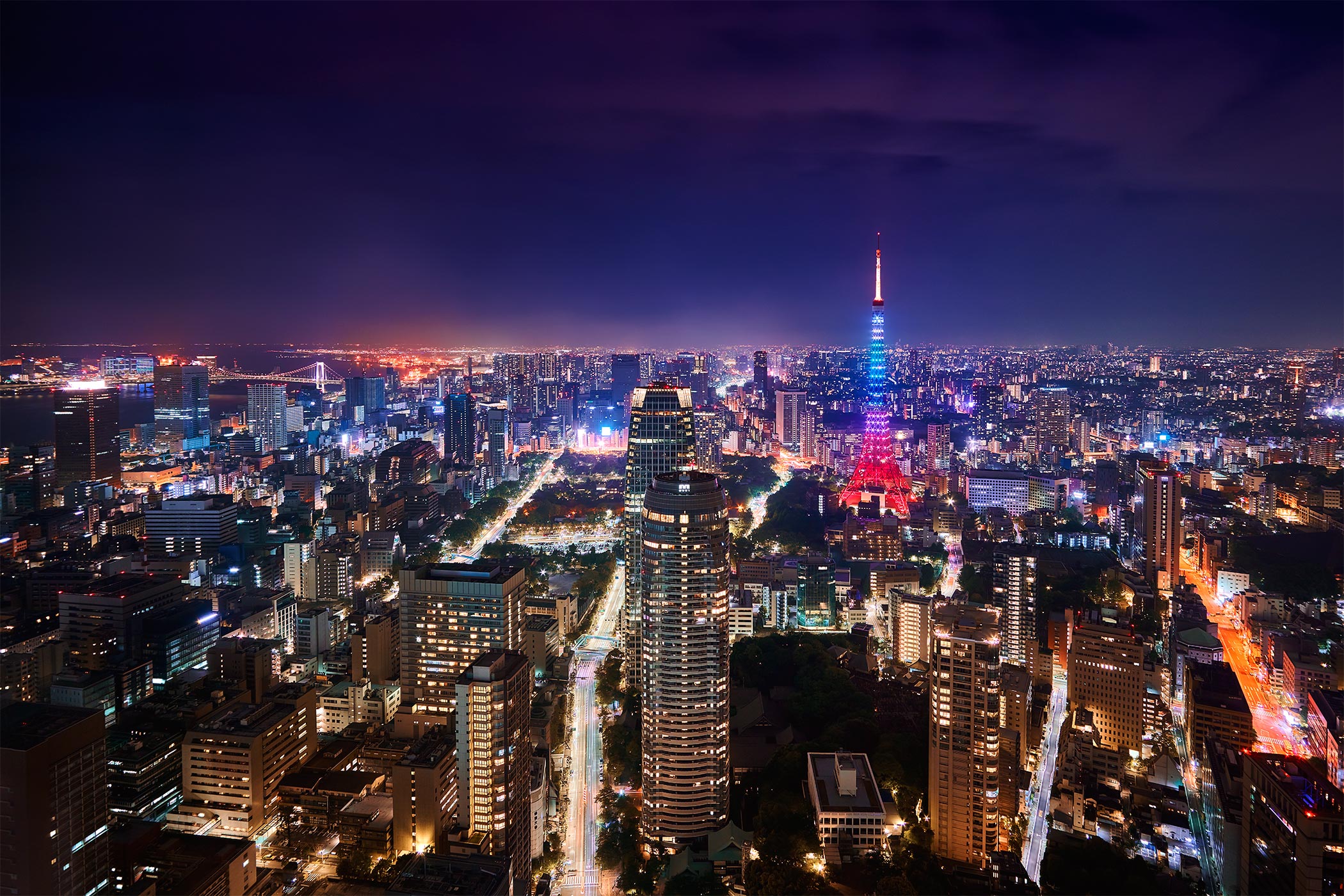An aerial nighttime photo captures the vibrant and bustling downtown of a large city, adorned with a striking tower in its center, reminiscent of both the Eiffel Tower and Tokyo Tower. The tower showcases a gradient of colors, illuminated red at the base, progressing to blue and white at the tip. This modern, slender structure is surrounded by high-rise buildings with brightly lit windows, contributing to the lively atmosphere of the city. The well-lit roads below are bustling with traffic, the cars forming streaks of light due to long exposure photography. The cityscape is speckled with a few trees along the sidewalks, but is predominantly an urban jungle. The night sky appears almost black, with hints of dark blue and faint clouds, the lack of visible stars a testament to the city's extensive light pollution. The entire scene exudes energy, creating a vivid representation of a thriving metropolis.